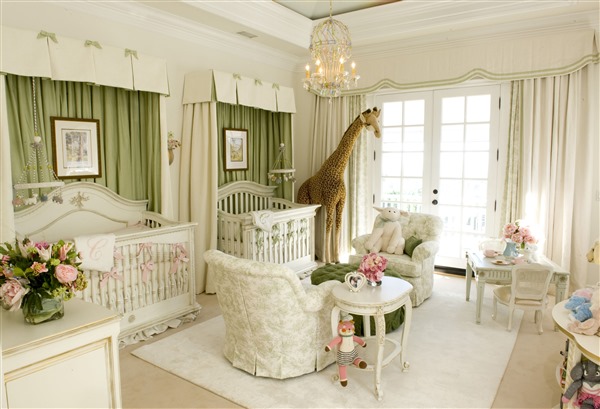This photograph showcases a luxurious and beautifully detailed baby nursery adorned primarily in white, exuding an air of elegance and sophistication. The room features white walls, white floors, and long white curtains with green trims that frame the French doors at the back. At the focal point of the nursery stand two intricately crafted white cribs with exquisite molding, each decorated uniquely with pink and green bows and matching monogrammed blankets with the letter 'C'. Suspended above each crib are delicate mobiles featuring pastel-colored animals, gently swaying to comfort the twins who presumably reside here.

The nursery's decor includes a plush green ottoman encircled by two overstuffed white chairs with a green pattern, creating a cozy seating area adorned with a white throw rug beneath it. Nearby, a side table holds a heart-shaped frame and a pink floral arrangement, while the room is further embellished with detailed crown molding and an elaborate chandelier hanging from the ceiling, casting a warm glow with its numerous electric candlesticks.

A prominent feature of the space is the towering giraffe stuffed animal, almost seven or eight feet tall, standing regally next to the crib with green bows. Throughout the room, various baby items are thoughtfully arranged, including a small table set with a child-size tea set and chairs, emphasizing the room’s charm and playfulness. Completing the elegant design is a white dresser adorned with gold trims and topped with another bouquet of pink flowers, adding a soft touch to the nursery's sophisticated ambiance. Enhancing the room’s visual appeal are two framed artworks hanging above each crib, the subjects of which remain unspecified, yet they contribute to the room’s intricate detailing and overall aesthetic beauty.